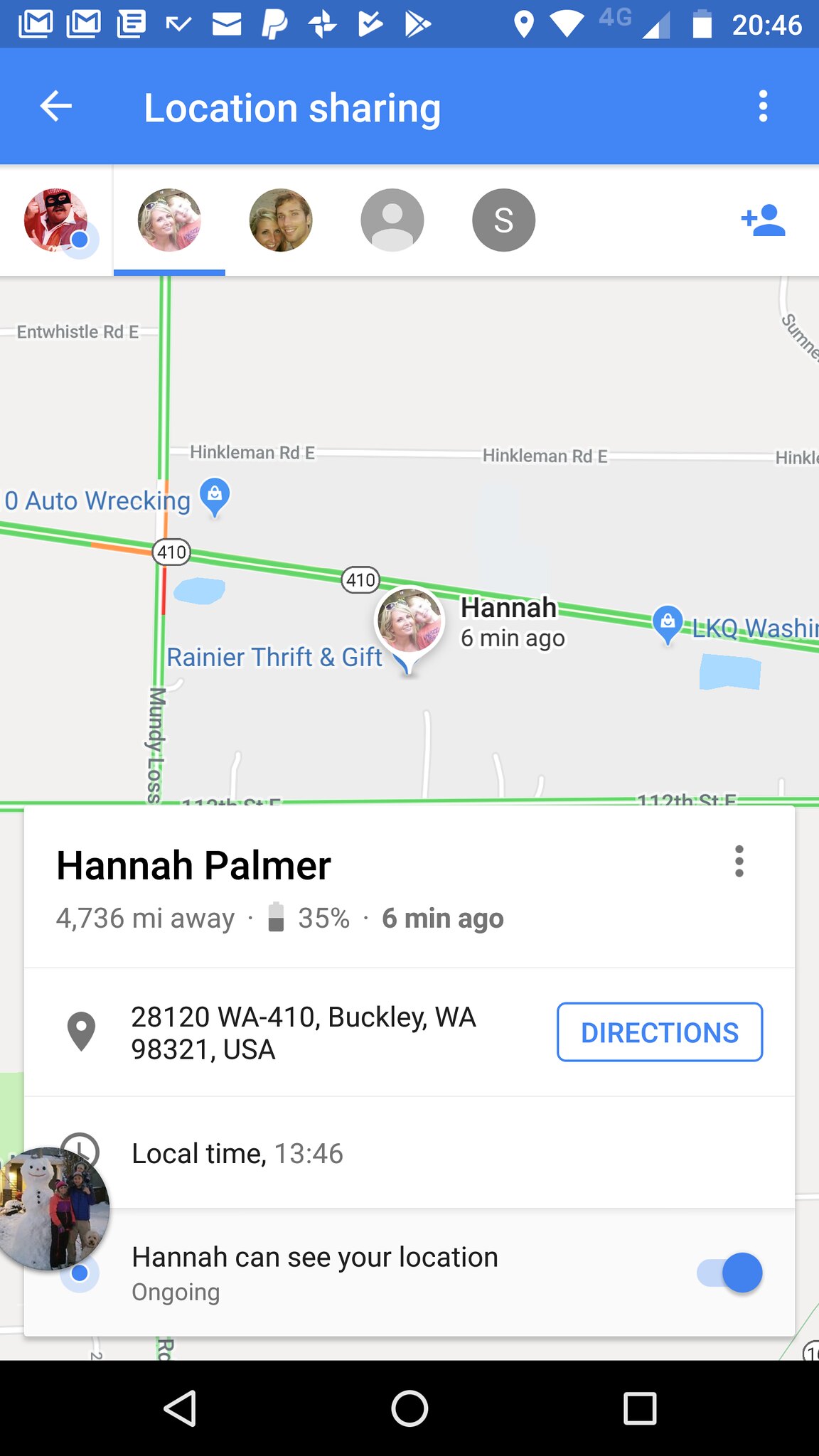This is a detailed screenshot of a Google Maps page displaying location sharing information. The image shows the user searching for an individual named Hannah Palmer, who is located 4,736 miles away. The interface prominently features a set of directions to Hannah's location. At the top of the screen, standard cell phone notifications are visible, including notifications for email, PayPal, and a Play Store update. The status indicators display full signal bars and battery level, and the clock shows the time as 20:46 in military time.

Just below the notifications, the blue text reads "Location Sharing," further specifying the context of the map. The main portion of the screenshot features a large, detailed map with Hannah Palmer's picture pinned to a specific road, indicating her exact location. The map has a white background with green lines clearly delineating various roads. The overall clean interface uses white text and icons for clarity.